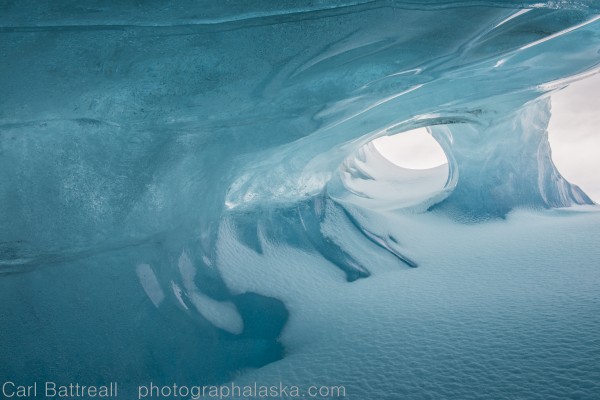In this captivating rectangular photograph taken outdoors during the daytime, we are presented with the stunning interior of an ice cave. Dominating the scene is a majestic ceiling of blue ice, swirling with darker blue patterns interspersed with white streaks. The curved wall and ceiling structure extend from the lower left-hand corner, sweeping up to the upper left and across to the right-hand side, before angling back down in a gentle curve.

On the bottom right portion of the image, we see a rippled, light blue-white snowy ground, resembling dimpled snow reminiscent of the patterns water forms in a water cave. This snowy surface starts just left of center and fans out to the lower right and then back towards the center, creating a delicate and serene effect.

A prominent detail on the right side of the photograph is an ice column descending from the ceiling, flanked by open spaces to its left and right, adding depth and framing the lower portions of the cave’s interior.

In the lower left-hand corner, against the vibrant blue ice background, the photographer's name, "Carl Battreall," is elegantly inscribed in white letters. Just to the right of his name, the caption reads "PhotographAlaska.com," providing credit and a hint of where to find more of his stunning work.

This detailed view perfectly captures the ethereal beauty and intricate textures of the ice cave’s interior.